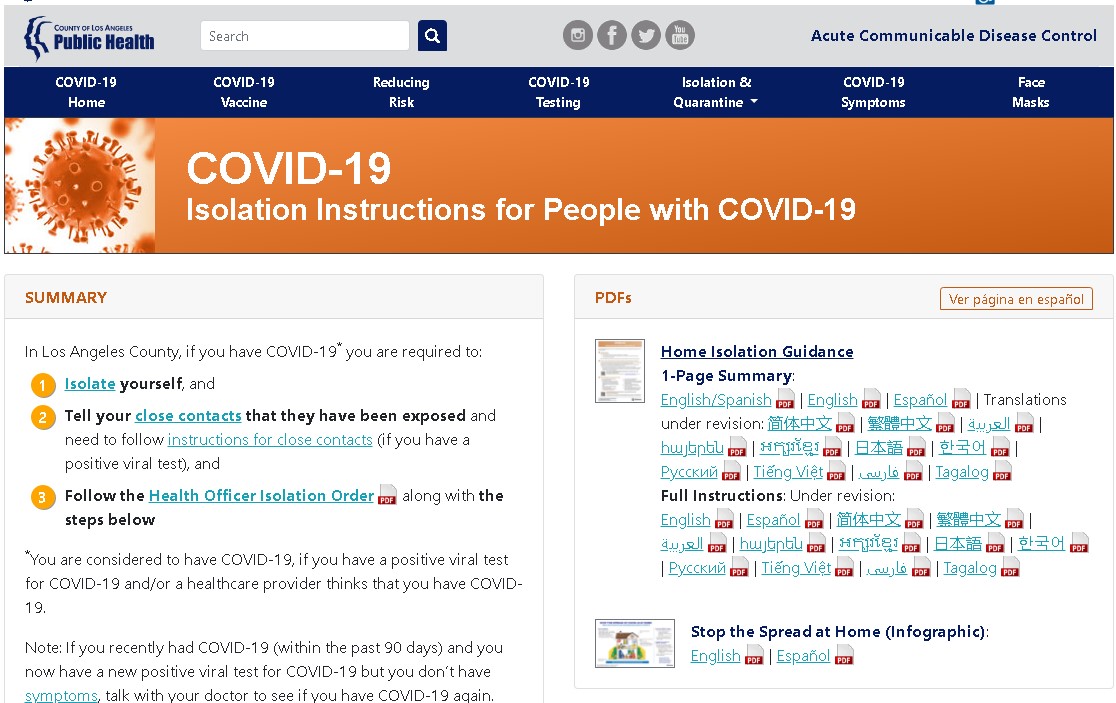An annotated snapshot of the Los Angeles County Public Health website is displayed. At the top, a horizontal gray bar spans the width, prominently featuring "Public Health" in the top left corner alongside a logo. To the right of the text is a search bar and search button. In the top center, social media icons for Instagram, Facebook, Twitter (or X), and YouTube are visible. In the upper right corner, the title "Acute Communicable Disease Control" is displayed.

Beneath this, a blue navigation bar stretches across, listing various COVID-19 related resources: "COVID-19 Home," "COVID-19 Vaccine," "Reducing Risk," "COVID-19 Testing," "Isolation and Quarantine," "COVID-19 Symptoms," and "Face Mask."

Below this blue bar is an orange section titled "COVID-19 Isolation Instructions for People with COVID-19." To the left of this section, there is a box labeled "Summary," containing more detailed information. To the right, several PDF links are provided, including "Home Isolation Guidance" and "Stop the Spread at Home Infographic."